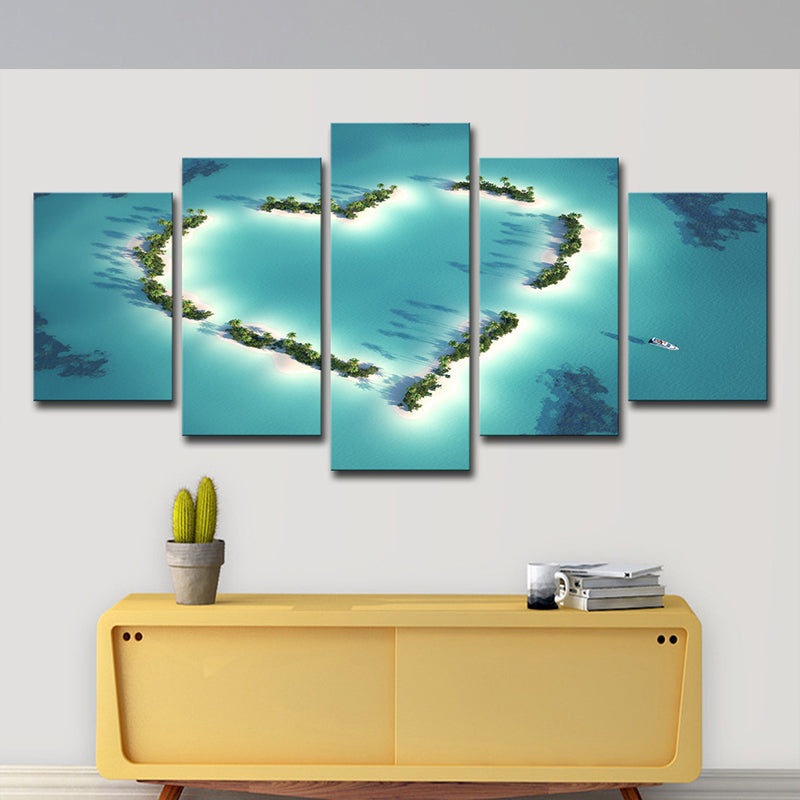The image showcases a modern, well-designed office scene. Central to the composition is a light-colored wooden credenza with two sliding doors that feature gold finger holes. Atop the credenza on the left side sits a gray pot containing a cactus with two upright, cucumber-like segments. To the right, there is a neat stack of thin books accompanied by a black and white mug. Above the credenza, five distinct panels are arranged artfully; they combine to form a cohesive scene of an island shaped like a heart, nestled within a body of water. The panels' predominant hues are varying shades of blue, accented with greens and touches of white and tan, portraying a serene overhead view that suggests islands and some greenery. The entire setting is illuminated with natural light, adding to the modern and airy atmosphere of the space. The wall behind the artwork is a light gray, complementing the white baseboard, and emphasizes the crispness and clarity of the overall design.